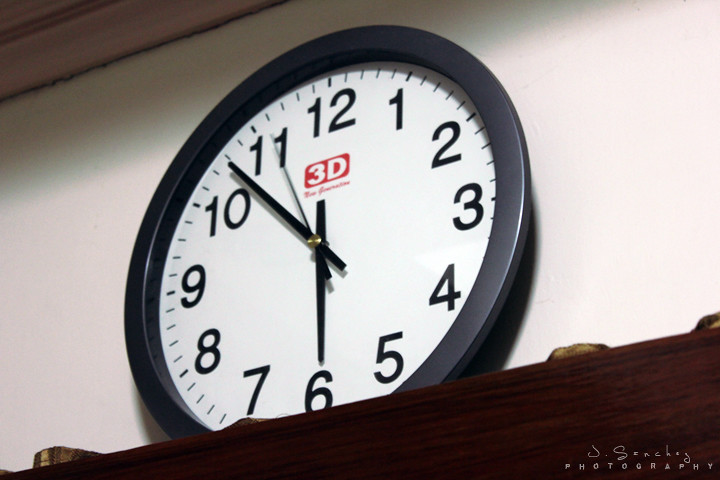This colour photograph features a round clock prominently displayed on a dark wooden shelf, positioned towards the bottom right corner of the image. The shelf exhibits several notches, adding a rustic charm to the scene. The clock, resting on the shelf rather than mounted on the wall, has a black rim and white face with black numerals marking each hour from 1 to 12. The clock hands are arranged with the large hand pointing between 10 and 11, the small hand at 6, and a tiny second hand directed towards 11. Behind the clock, the wall is a beige hue, with shadows enveloping the upper section, particularly the top left corner, suggesting a subtle interplay of light and shade. In this top left corner, there is an additional wooden element—possibly another shelf, frame, or part of the roof—running diagonally, hinted by a visible plank of wood. Adding a finishing touch, in small white script just beneath the shelf, is the signature "J. Swankie" or "Swankie Photography," denoting the artist or photographer responsible for the image.